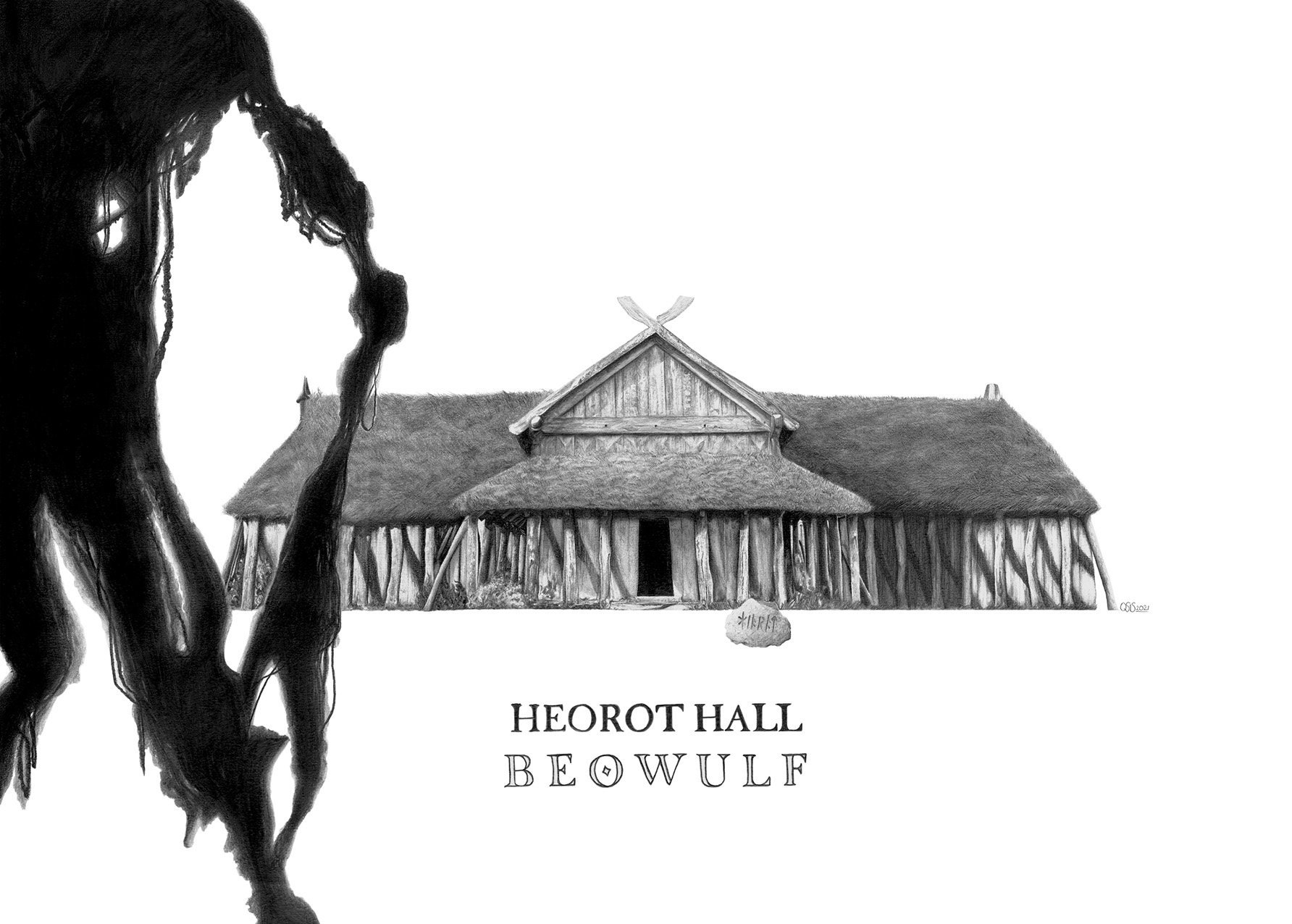This black-and-white drawing depicts a large building identified as "Heorot Hall," a significant setting from the epic Beowulf, inscribed in bold black letters with the word "Beowulf" beneath it in thin white lines. The building in the background appears to be a grand, communal Viking hall characterized by its wooden structure, prominent pillars, and possibly a thatched roof. This hall, a civic center for the village, serves as a central gathering place for communal meals and other activities. The foreground features an eerie element—a long, ragged, black figure or creature that could represent the legendary characters Beowulf or Grendel, approaching the hall. This creature appears almost spectral, with thin, moss-like lines trailing from it, adding a mysterious, haunting atmosphere to the scene. The detailed texture of the drawing suggests it might be rendered in charcoal, enhancing the stark contrast and intricate design of both the building and the enigmatic figure.